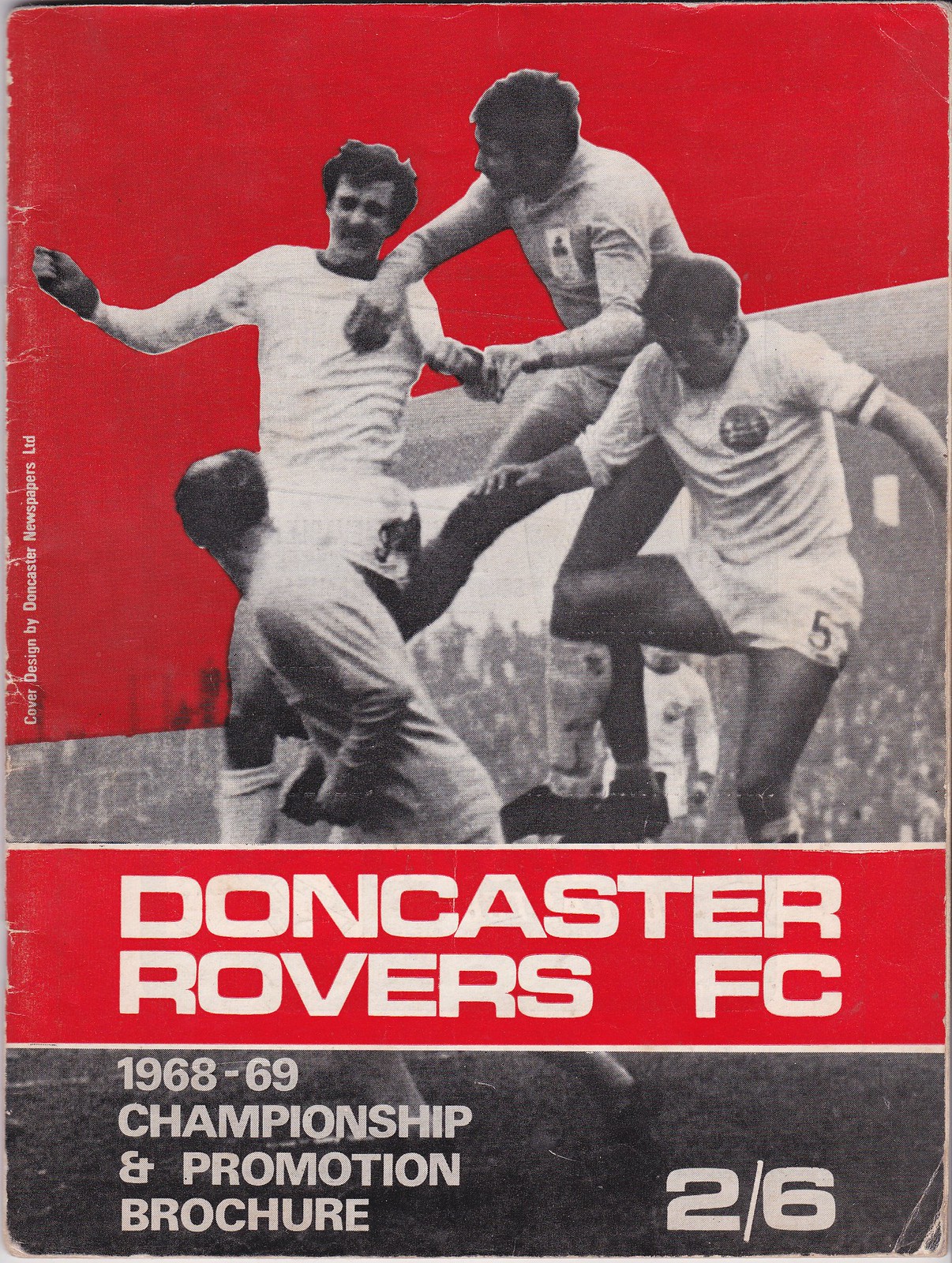This image is a vertically aligned, aged magazine cover or brochure, showcasing a soccer theme. Prominent wear and tear on the left-hand side spine displays small rips and creases, indicating it is an old item from the late 1960s. The top of the background is red, transitioning to gray in the middle, with alternating red and gray bands at the bottom. 

At the upper portion of the cover, there's a black-and-white photograph capturing four soccer players mid-air, all dressed in long-sleeved white shirts and white shorts. The background features a blurry stadium and stands filled with spectators. Just below this image, a horizontal red banner with large, white, all-capital letters reads "DONCASTER ROVERS FC".

Further down, the background turns gray and black, resembling grass under the players' feet. On the bottom left of this section, gray text reads "1968-69 Championship and Promotion Brochure." In the lower right-hand corner, a bold number "2/6" is visible. The overall quality of the image is low, characteristic of the print design of that era, with visible dots and signs of aging such as creases and worn paint.